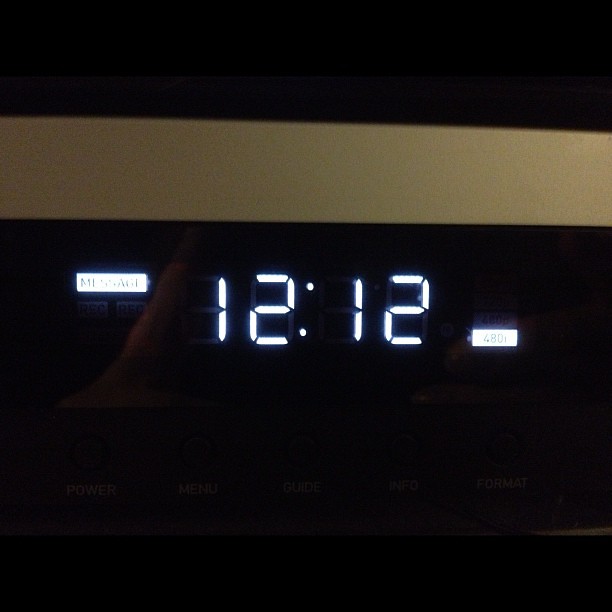A detailed close-up view of a digital faceplate on what appears to be a television receiver or cable box. The faceplate features a prominent rectangular black digital display. In the top left corner, there is a small rectangle labeled "Message." In the bottom right corner, a tiny rectangular indicator displays "480p," likely denoting the resolution format. The digital clock in the center of the display reads "12:12" in bright, legible numerals. Along the bottom of the faceplate, several functional buttons are neatly labeled: "Power," "Menu," "Guide," "Info," and "Format." The uppermost part of the image fades into a solid black background, drawing attention to the illuminated details of the faceplate.